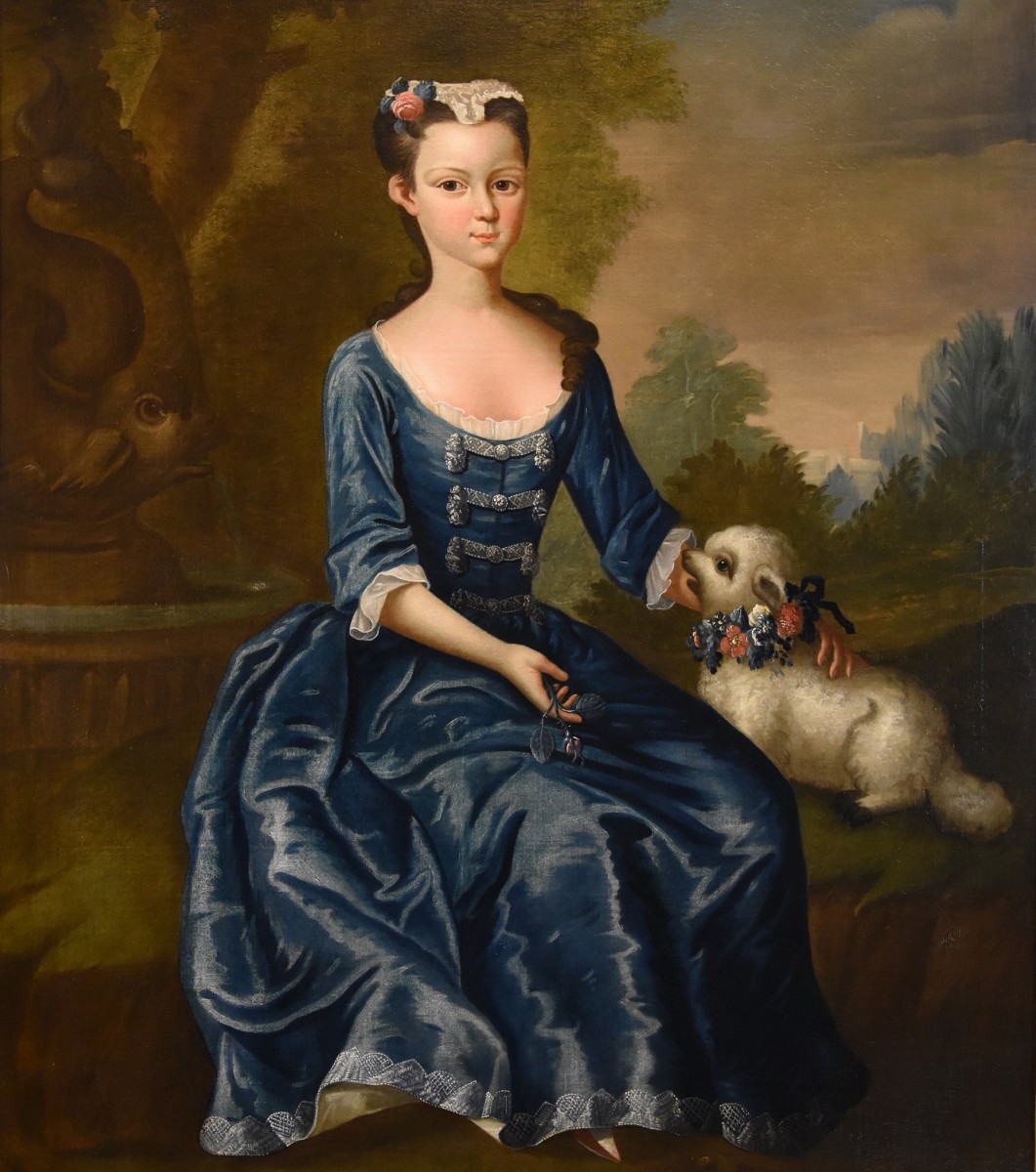The painting portrays a young girl from the Victorian era, dressed in an elaborate navy blue gown made of shiny material. Her brown, curly hair is partially pulled back, some of which cascades over her left shoulder. She wears a flowered hairpiece that resembles a doily. Standing to her right is a small, white, curly-haired dog adorned with a floral necktie featuring both blue and pink flowers. The background suggests she is situated in front of a garden, with some trees and a water fountain shaped like a statue, potentially depicting a fish, spouting water on the left side of the painting. The setting appears to be during twilight, adding a dim, serene atmosphere to the scene.